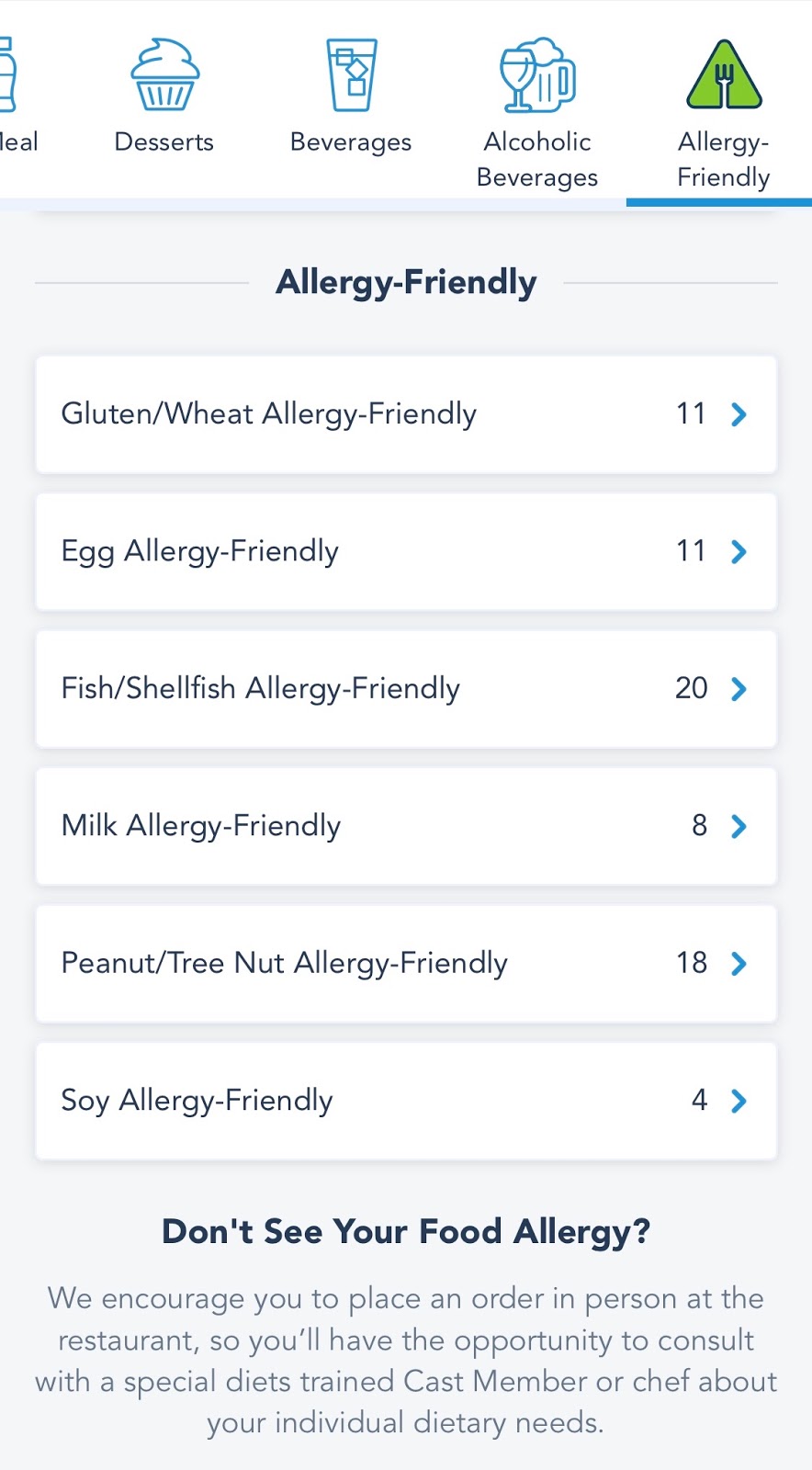This image, taken from an app, is meticulously divided into several sections to guide users through its various features. 

At the top, there are distinct icons representing different categories: desserts, beverages, alcoholic beverages, and allergy-friendly options. 
- The desserts category is illustrated with a cupcake icon.
- The beverages category features a glass with ice cubes in a blue-lined outline.
- The alcoholic beverages category is depicted with icons of a wine glass and a beer mug.
- The allergy-friendly category is marked by a fork within a green triangle.

Below this section, the app emphasizes the allergy-friendly options with a prominent heading followed by a menu icon that lists "gluten, wheat, allergy-friendly" dishes, marked with an '11' and a button to continue.

Further down, the app lists additional allergy-friendly categories, each marked with a clickable blue arrow for more information:
- Egg Allergy-Friendly
- Fish & Shellfish Allergy-Friendly
- Milk Allergy-Friendly
- Peanut & Tree Nut Allergy-Friendly
- Soy Allergy-Friendly

Finally, at the bottom, the app provides a recommendation for users who have dietary restrictions that may not be covered by the listed categories. It encourages them to place their orders in person at the restaurant to consult with a special diet-trained cast member or chef about their individual dietary needs.